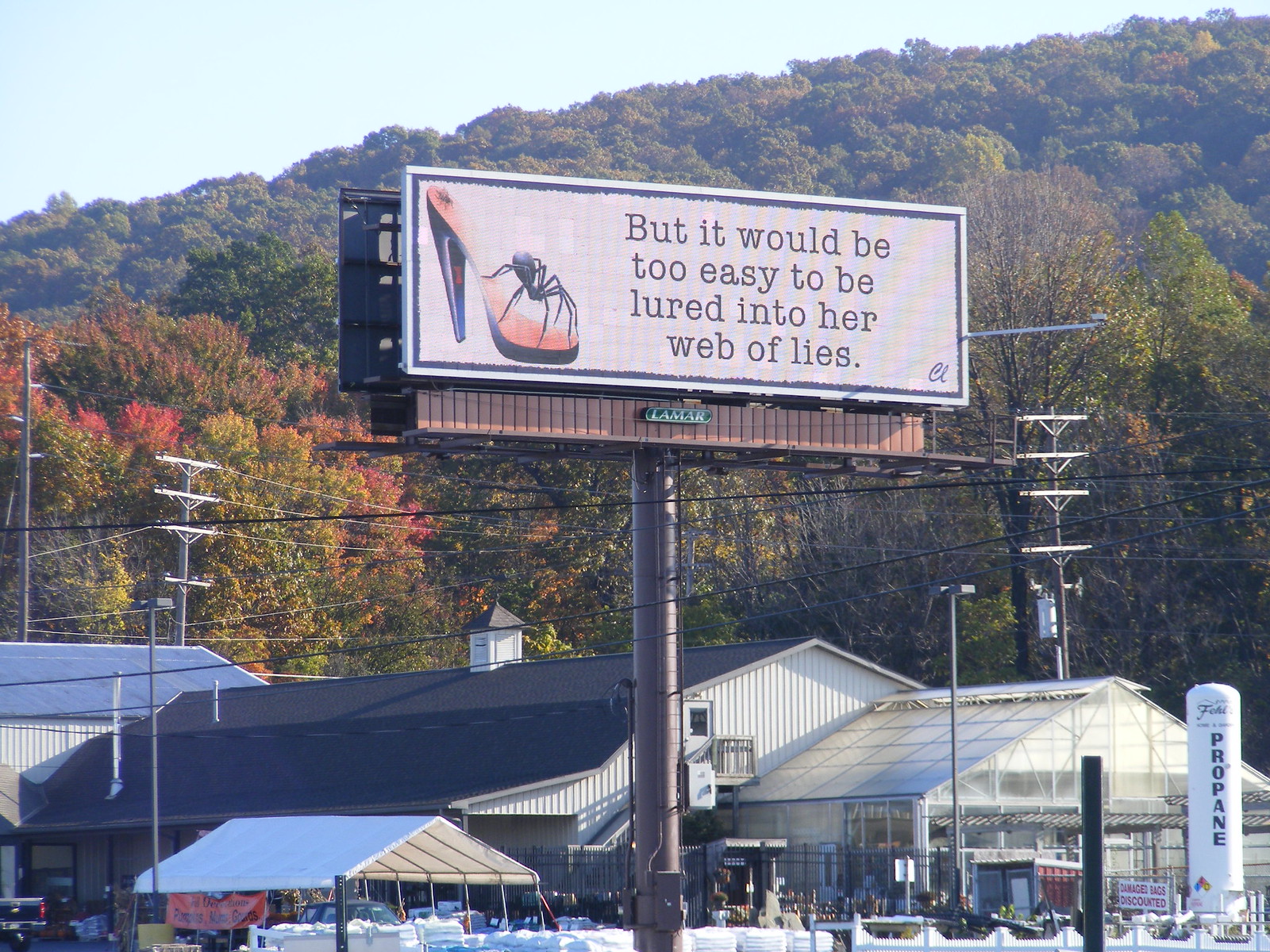The photograph showcases a prominent billboard centrally mounted on a dark brown metal pillar, positioned in front of a large building resembling a metal barn or warehouse, with a greenhouse extension on the right. Below the billboard, there is a parking lot featuring a canopy tent and pallets of plastic-wrapped items. To the lower right, a white propane tower is visible, bearing the word "propane." The billboard itself has a light tan background and is bordered in black. It prominently displays a striking image of an orange-colored high heel with a tall black stiletto heel, and a large black widow spider perched on the front part of the shoe. To the right of this image, centered in black text, the billboard reads, "but it would be too easy to be lured into her web of lies." The background includes hills covered in dense foliage, with trees showing vibrant autumn colors of red and orange mixed with green. Power lines stretch across the scene, adding to the detailed backdrop.